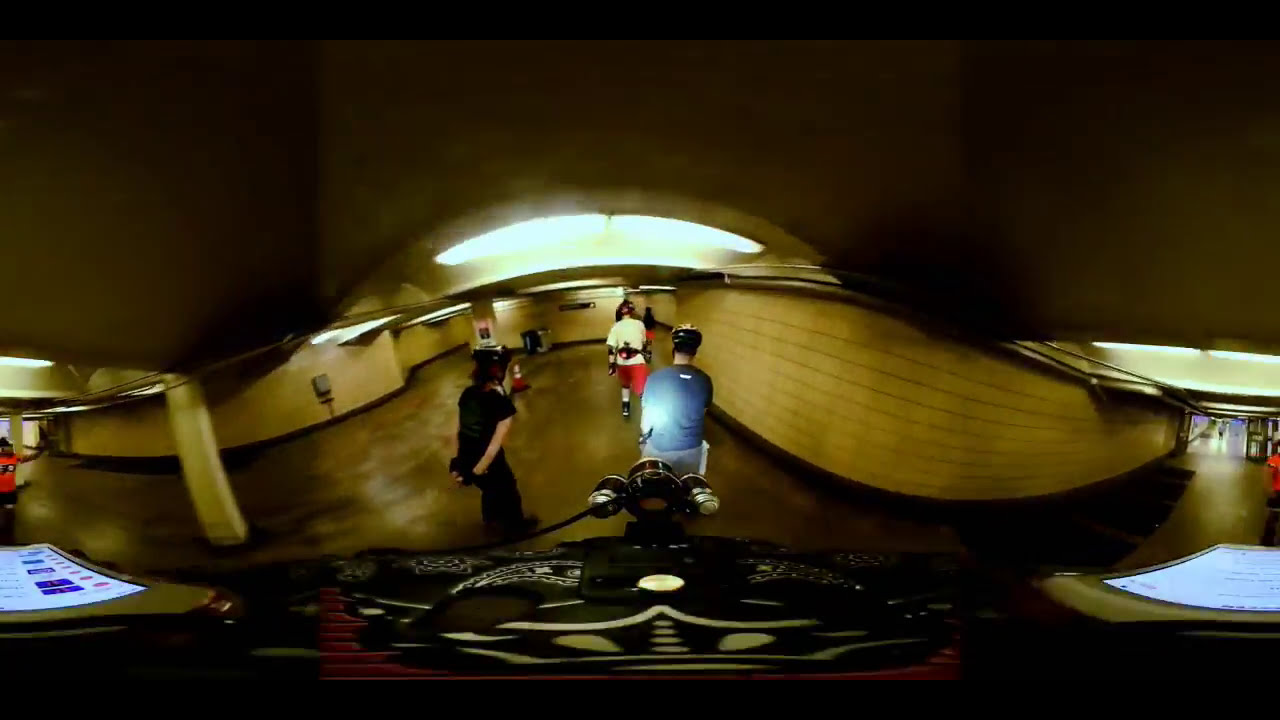The image appears to be a distorted panorama, possibly from a security camera or a dashboard recorder, taken in a parking garage or a roller rink-like space with curving walls and odd shadows creating a fish-eye lens effect. The scene is characterized by a dark brown, curved archway with lights overhead, and a beam extending to the ceiling. In the foreground, there is a peculiar black, white, and red area with white dots and a red border. On the far left, a person in an orange shirt stands near a car, while on the right side, there's another car and a hallway leading to a brightly lit doorway. The middle of the image is dominated by three young men: one in a black outfit with wrist pads and both hands behind his back, another in a blue shirt and black helmet, suggestive of skaters, all wearing helmets. The ground and borders of the image have a noticeable curve, indicating a panoramic distortion.